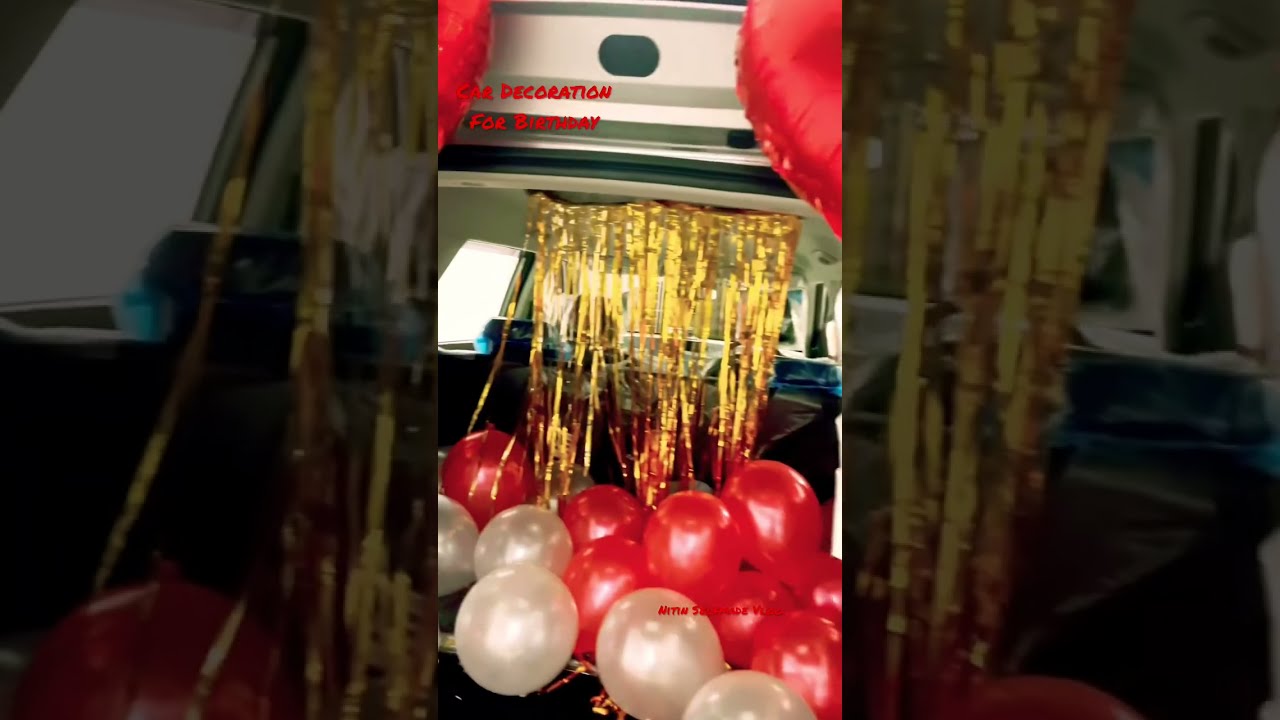The image depicts the inside of a vehicle, possibly a car or camper, decorated for a birthday celebration. Golden streamers hang from the ceiling, obscuring the view of the blue-colored seats in the background. Red and white balloons are scattered across the floor and appear at the top corners of the image, some of which seem heart-shaped. The windows of the vehicle are visible, adding to the sense of interior space. At the top of the picture, a small caption reads "Car Decoration for Birthday," while at the bottom, red text spells out "N-I-T-I-N" with additional words obscured by red-on-red balloon placement. The overall image is lively and festive, enhanced by a partially transparent, blown-up version of the same scene in the background.